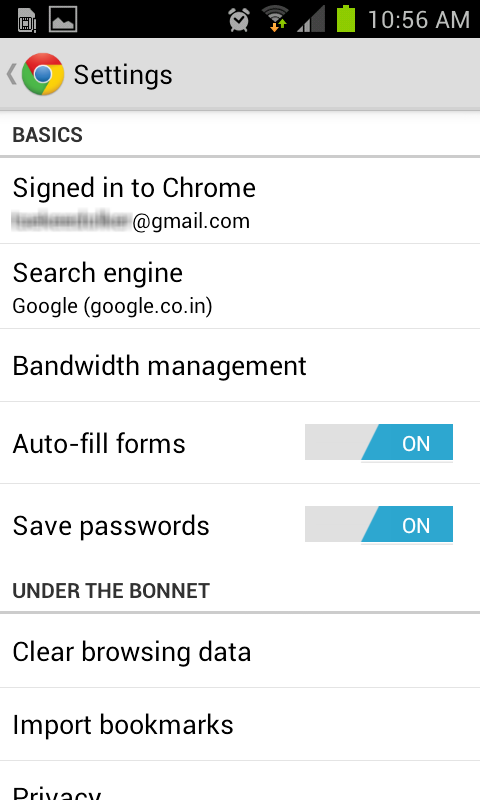Screenshot of a mobile device displaying the Google Chrome settings page. The top section of the screen features a black status bar that includes several phone indicators. On the far right, it displays the time "10:56 AM", a green battery icon, signal strength bars, Wi-Fi signal icon, and an alarm clock symbol. On the far left, there are icons resembling an SD card or SIM card, and a mountain image, possibly indicating an active photo or file transfer.

Below the status bar, the user is navigated to the "Settings" section of Google Chrome. The Chrome logo is visible at the top, followed by a category labeled "Basics." Under this category, it shows that the user is signed into Chrome with their email address displayed. The "Search engine" is set to "google.co.in". Further down, there are options such as "Bandwidth management" and "Autofill forms," the latter of which has a toggle switch that is half-gray and half-blue, indicating it is turned on. Below this, there's a "Save passwords" option, also switched on with a similar toggle button.

The "Under the bonnet" section follows, offering options like "Clear browsing data" and "Import bookmarks." The word "Privacy" is partially visible at the bottom, indicating more options may be available but are cut off in the screenshot. This image depicts a user adjusting their settings within the Google Chrome browser on their mobile phone.